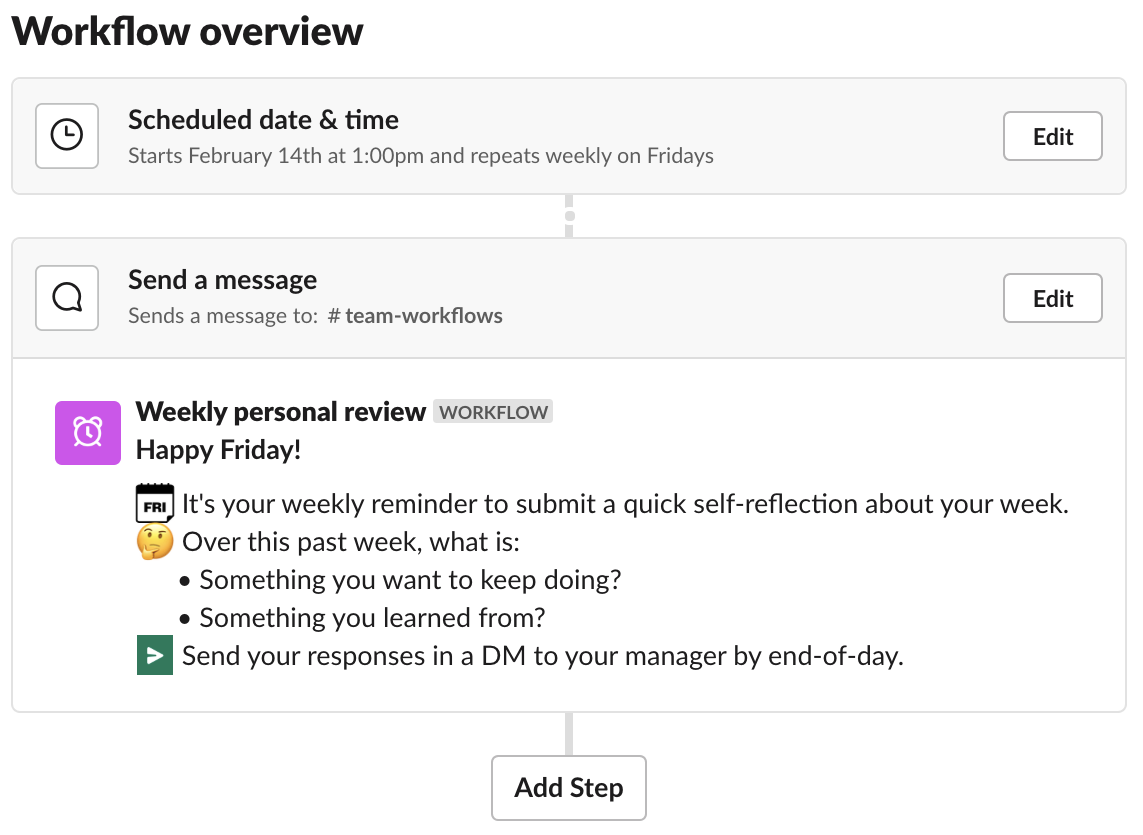The image presents a detailed workflow overview set against a primarily white background. 

In the upper left section, there is an area titled "Workflow Overview." Beneath this, the first rectangular gray box displays the following schedule details: "Start: February 14 at 1 p.m.," and "Repeats weekly on Friday." To the right of this box, there is a gray button labeled "Edit" in black font.

Below this, another elongated gray rectangle contains the instruction: "Send a message to #team-workflows." Adjacent to this, another gray "Edit" button appears.

Continuing down, on a white background, the section titled "Weekly Personal Review Workflow" offers further details. It reads: "Happy Friday! It's your weekly reminder to submit a quick self-reflection about your week. Over this past week, what is:" followed by bulleted points: "Something you want to keep doing," and "Something you learned from." Below these points, a green box with a white right arrow instructs, "Send your responses in a DM to your manager by the end of the day."

At the very bottom, a white button with black text invites the user to "Add Step." 

To the right of the "Weekly Personal Review Workflow" heading, a purple square bearing a white alarm clock icon is visible. The header text "Weekly Personal Review Workflow" is in gray with "WORKFLOW" highlighted in uppercase below.